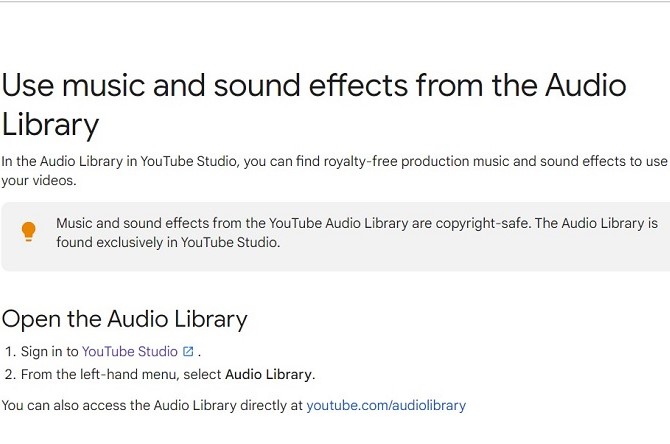This image is a screenshot of a section from an audio website, presumably YouTube Studio, displayed on a predominantly white background. The portion seems cropped, indicating it is a fragment of a larger page. 

At the top of the screenshot, bold black text reads, "Use Music and Sound Effects from the Audio Library." Beneath this, smaller gray text provides further details: "In the audio library in YouTube Studio, you can find royalty-free production music and sound effects to use in your videos."

Following this, a gray rectangular box stretches across the screen, containing a yellow light bulb icon on the left. Inside the box, black text states, "Music and sound effects from the YouTube Audio Library are copyright safe. The audio library is found exclusively in YouTube Studio."

Below this, slightly larger black text directs users to "Open the audio library." 

A step-by-step list is provided underneath, guiding users on how to access the audio library:
1. Sign into YouTube Studio.
2. From the left-hand menu, select Audio Library.

It also mentions that the audio library can be accessed directly at youtube.com/audiolibrary.